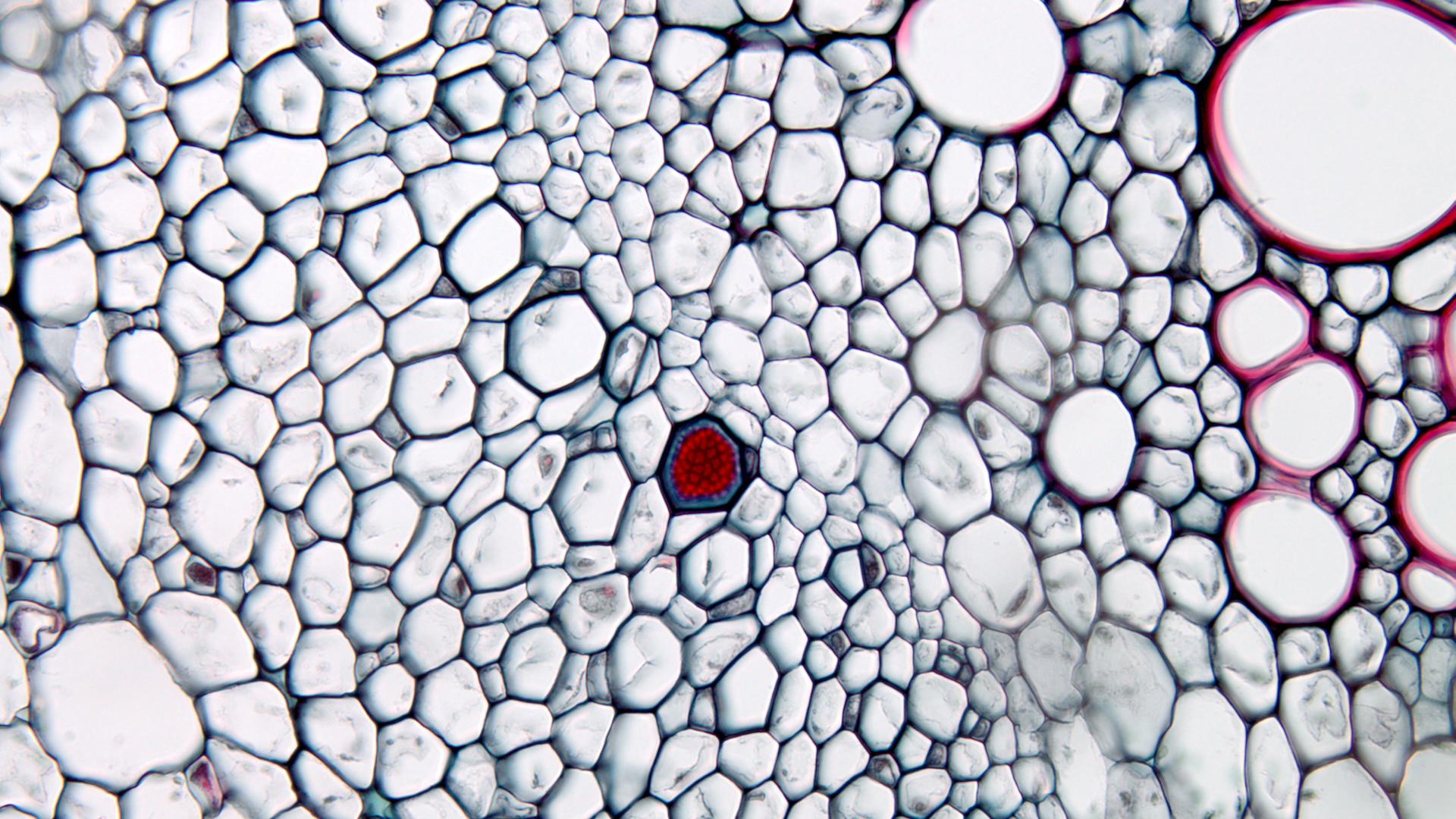This image features a close-up view of a detailed and intricate artwork composed of numerous tiny pebbles arranged in various patterns. At the center of the photograph, white pebbles are meticulously organized to create a beautiful, flower-like design. To the left of this central motif, additional white pebbles are neatly aligned, creating a harmonious contrast. Just above these pebbles, a single brown pebble with blue outlines stands out, adding a unique detail. To the right of the central flower pattern, larger pebbles with striking white centers and red edges offer a bold visual impact. The overall composition is quite striking, with the white pebbles forming elaborate floral patterns throughout the artwork. This intricate arrangement suggests that it might be part of an art exhibit, showcasing the meticulous use of pebbles to create elaborate designs.